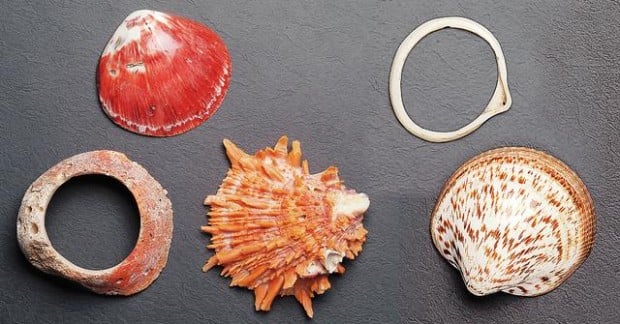The image features a collection of five seashells displayed on a dark gray surface. The top left shell is predominantly red with a glossy, smooth finish, bordered in white, and features a white underside. Directly below it is a shell with a professionally smooth, hollow center, almost as if it had been drilled. Adjacent to this is an intricate, spiny orange shell, notable for its rough texture. To its right, there's another seashell with a white base, speckled with brown flecks, and it has a rounded, smooth appearance. Above this last shell is another hollow, ring-shaped shell, slightly thicker and containing shades of brown and reddish hues. The meticulous arrangement and variety of textures and colors make the photograph both visually engaging and detailed.